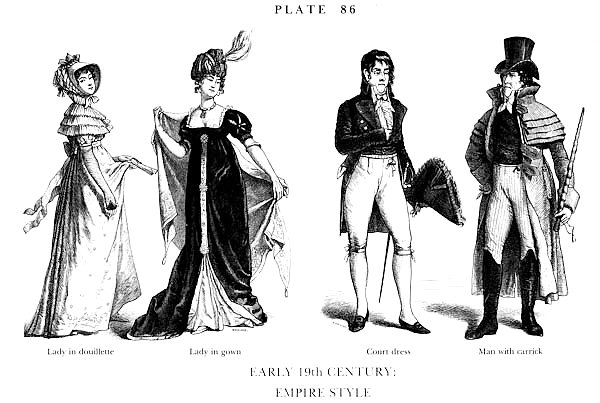This image features detailed sketches of four individuals adorned in early 19th century Empire style attire, likely derived from a historical book or poster. At the top of the image, it is labeled "Plate 86" and at the bottom, it reads "Early 19th Century Empire Style." The background is predominantly white, directing focus to the central figures who are rendered in shades of black, white, and gray. 

On the left, a lady stands in a dowelette or jubilee, her attire characterized by the fashion conventions of that period. Next to her is another lady attired in a formal gown. The first gentleman to the right of these two women is dressed in a court (or count) dress, complete with pants and a long tailcoat, embodying the distinguished style of the era. The final figure on the far right is a man holding what appears to be a carrack or kirk, which resembles a cane, and he is adorned with a top hat. This compilation of figures, with two women on the left and two men on the right, offers a window into the sartorial elegance of the early 19th century, capturing the textures and nuances of Empire style fashion.